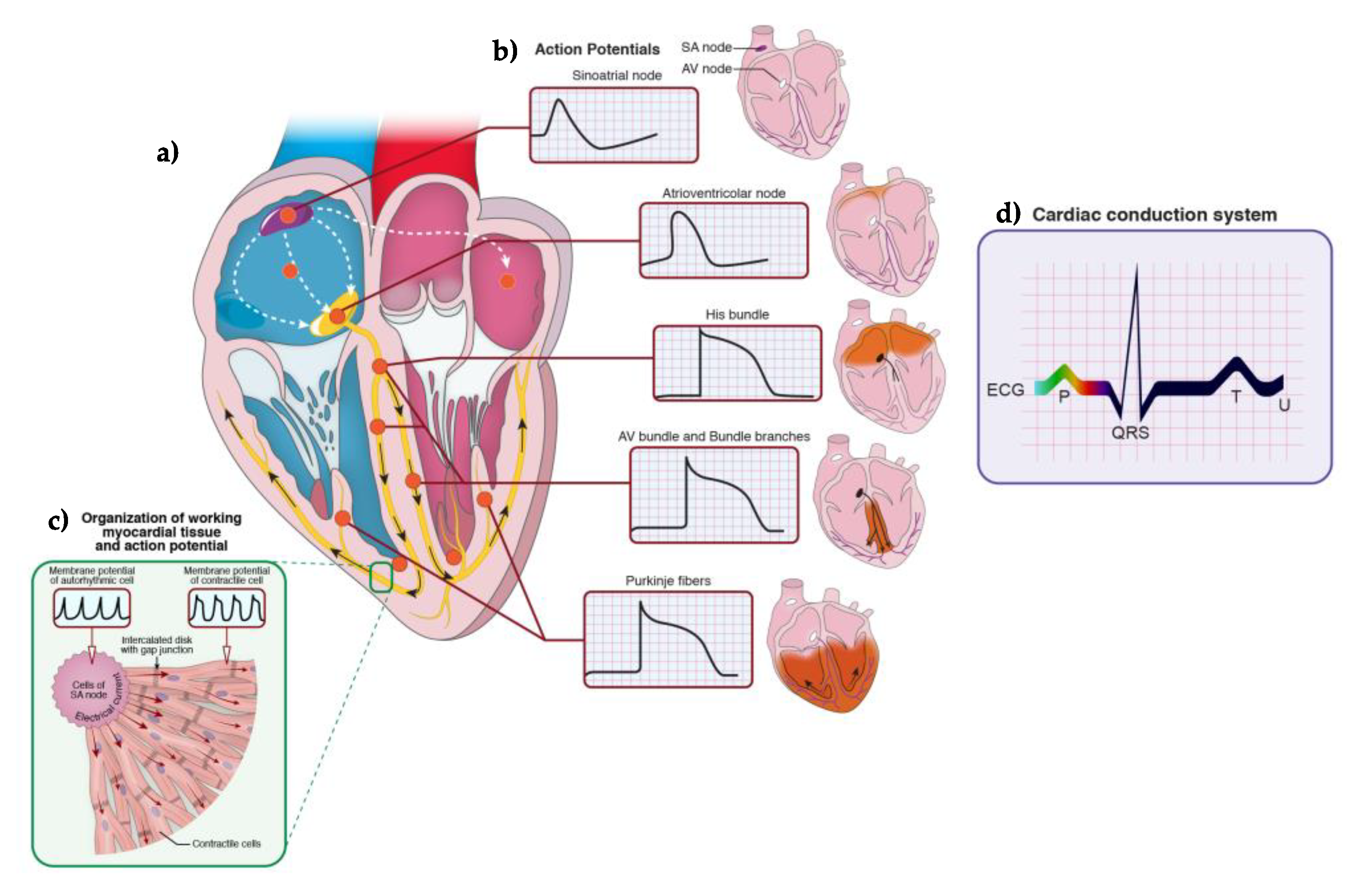This detailed horizontal medical diagram illustrates the intricate workings of the human heart, most likely sourced from a medical instructional book. Prominently, the diagram features a cross-sectional cutout of the heart in the upper left corner, vividly displaying its various chambers and key components such as the SA (sinoatrial) node and AV (atrioventricular) node. Adjacent to this heart illustration, there are several smaller diagrams that depict the electrocardiogram (ECG or EKG) readings for each heart chamber, carefully detailing the blood flow and electrical signals that characterize a heartbeat.

Below these diagrams, additional explanatory text further delves into the specifics of heartbeat signaling, although some parts of the text are not clearly legible. On the right side of the image, a colorful and detailed ECG graph highlights the electrical activity of a single heartbeat, with distinct colored lines (green and blue) corresponding to various phases of the cardiac cycle. This section includes labeled peaks and troughs, with annotations such as A, B, and C to guide the viewer through the sequential steps of the heart's electrical activity. This comprehensive and visually appealing diagram provides a thorough overview of the heart's function, emphasizing the scientific principles behind cardiac physiology.